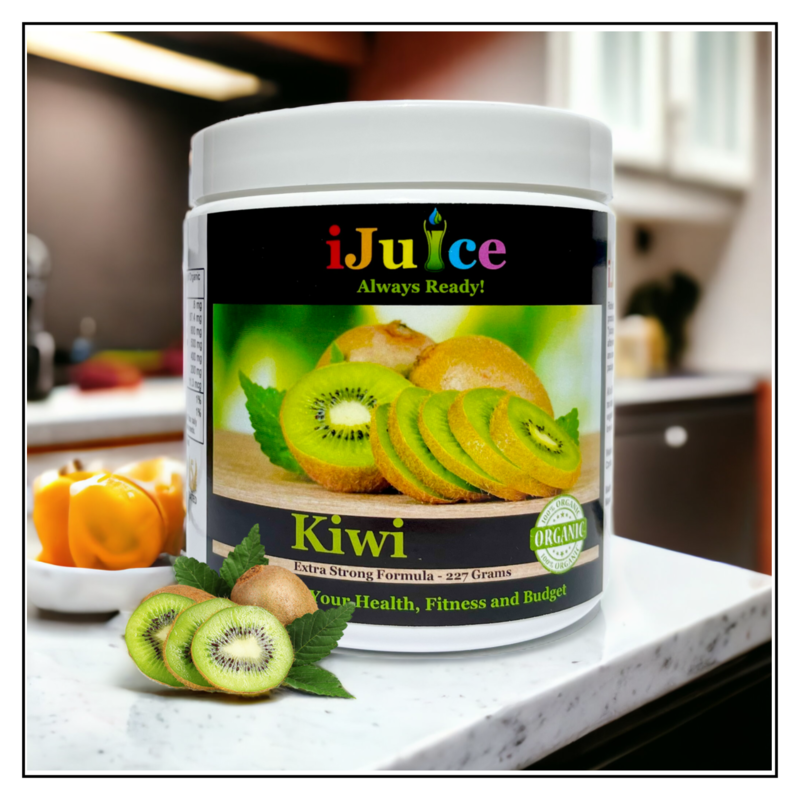This detailed photograph captures a nutritional product prominently placed on a white and gray speckled marble countertop in a kitchen with a blurred background showing some cabinetry and indistinct objects. The product itself is housed in a white plastic canister with a white lid. The canister features a distinctive black label that wraps around its surface. At the top of this label, the brand name "iJuice" is vividly displayed in text with letters alternating through the colors of the rainbow—red, orange, yellow, green, blue, and purple. The "i" in "iJuice" is stylized, shown as a glass filled with a green liquid, topped with a blue water droplet.

Beneath the brand name, the tagline "Always Ready" is written in green text. Dominating the central portion of the label is a large, vibrant picture of kiwi fruits. On the left, there's a half kiwi fruit clearly displaying its seeds and green flesh. Adjacent to this is another kiwi fruit sliced halfway, while two whole brown kiwis are positioned behind. Further down the label, in green text, the word "Kiwi" appears. Below this, a pink stripe features the text "Extra Strong Formula, 227 grams" in black. Additional green text at the bottom declares the product's benefits: "Your Health, Fitness and Budget." To the right of the kiwi image, a small white and green label with the word "Organic" is visible.

Complementing the canister, assorted fruit slices, including cut-up kiwis and a whole kiwi, are artistically arranged to the left, accompanied by a white bowl that is orange inside. The detailed imagery and vibrant text on the label emphasize the product's natural and health-focused attributes.